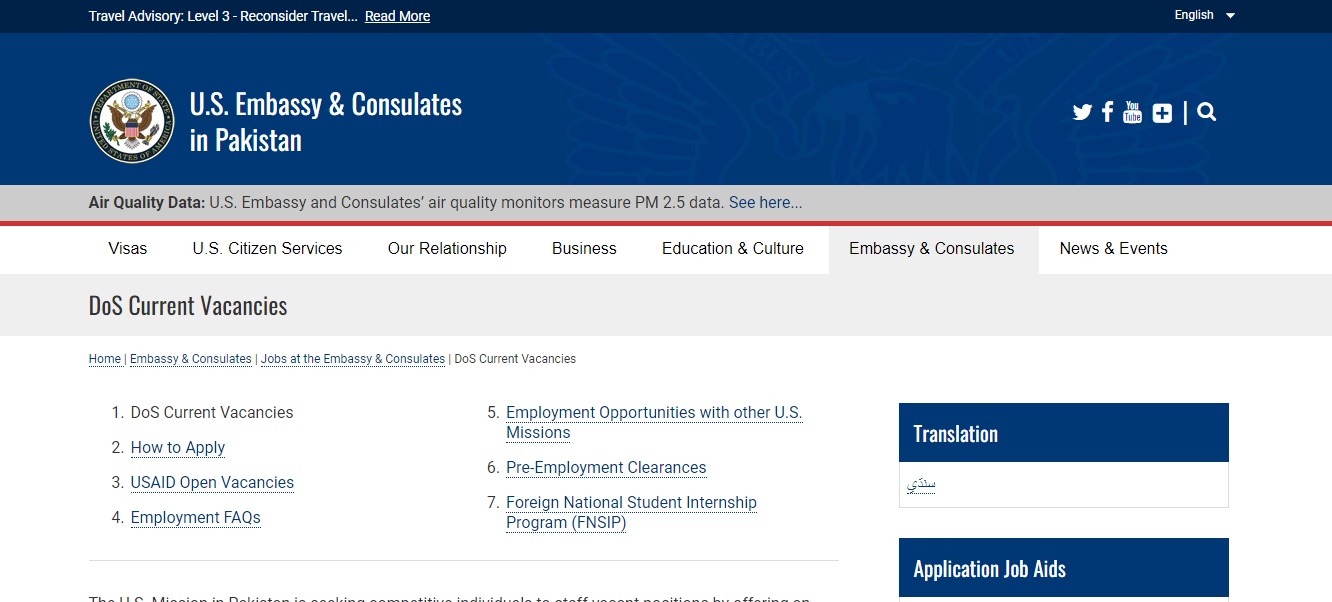The image showcases a detailed view of a website interface. At the very top, a navy-blue banner spans the width of the page, prominently featuring a travel advisory labeled 'Level 3 - Reconsider Travel', with an option to 'Read More'. To its right, a language selection drop-down menu appears, which currently only offers English.

Beneath this, a blue band displays the title 'U.S. Embassy and Consulates in Pakistan', accompanied by the official U.S. seal on its left. To the right of this title are icons for Twitter, Facebook, and YouTube, alongside a mysterious plus symbol which suggests additional options, and a search bar. 

The section immediately below reads 'Air Quality Data — U.S. Embassy and consulates air quality monitors measure PM 2.5 data'. This establishes the focus on air quality monitoring provided by the embassy and consulates.

Further down, various clickable sections are organized into categories: Visas, U.S. Citizen Services, Our Relationship, Business, Education and Culture, Embassy and Consulates, and News and Events. Currently, the 'Embassy and Consulates' section is selected, revealing further details about employment opportunities.

Under 'DOS, Current Vacancies', an abbreviation for the Department of State, a sub-menu lists home links such as 'Jobs at the Embassy and Consulates' and 'DOS Current Vacancies'. The section is divided into seven listed items: 
1. DOS Current Vacancies
2. How to Apply
3. USAID Open Vacancies
4. Employment Frequently Asked Questions
5. Employment Opportunities with Other U.S. Missions
6. Pre-Employment Clearances
7. Foreign National Student Internship Program

Additionally, a section for 'Translation and Application Job Aids' is available for those interested in employment with the Department of State (DOS).